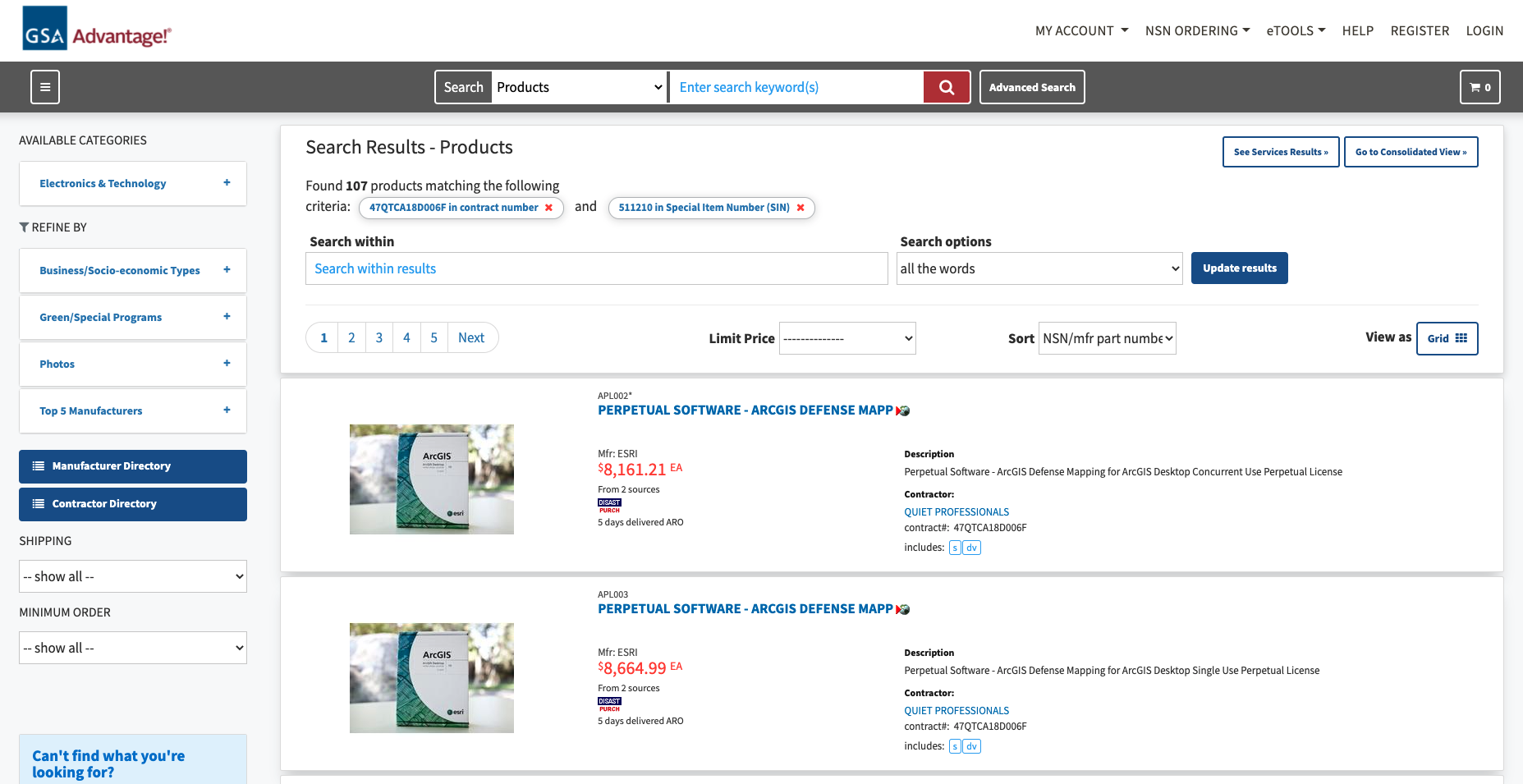Screenshot of the GSA Advantage Homepage

The image captures a screenshot of the GSA Advantage homepage, a government procurement website. On the left side of the page is a sidebar with a section titled "Available Categories," listing various categories like electronics, which users can refine based on their needs. The menu also includes options such as NSN ordering, e-tools, help, and the functionalities for registering or logging in.

The main interface has two distinct search areas: one for keywords and another for products, making it easier to locate specific items. The page features a predominantly white background with some elements in dark blue, giving it a clean and professional look. Notably, there is software listed for purchase, priced at $8,161, along with programs like defense mapping, indicating the specialized nature of the products available.

Designed for government contractors, the site outlines shipment details, minimum order requirements, and specific budget allocations. There is a prominent red search box marked by a magnifying glass icon, where users must log in to their accounts to initiate a search. This interface allows for streamlined purchases catering to the needs of government operations.